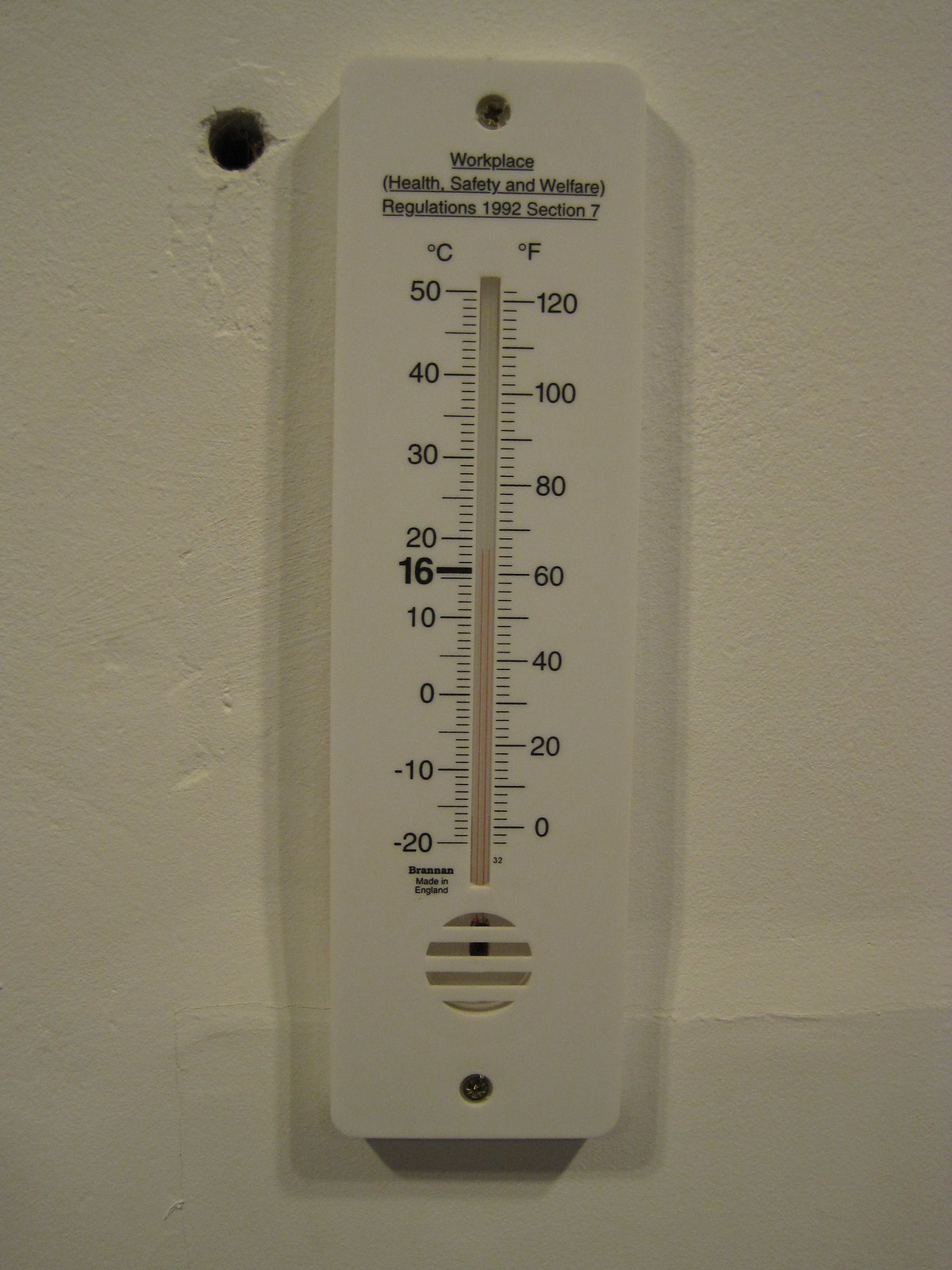The image features a white concrete wall with a prominently mounted wall thermometer. This thermometer has a long, rectangular shape with smoothly rounded corners and a sturdy white plastic casing. Detailed text is prominently displayed at the top of the thermometer in black, underlined letters, reading "Workplace Health, Safety, and Welfare Regulations 1992, Section 7." The thermometer displays temperature readings in both Celsius and Fahrenheit. On the left side of the scale, the Celsius measurements range from -20°C to 50°C, while on the right side, the Fahrenheit scale spans from 0°F to 120°F. The dual-scale design allows for a comprehensive understanding of temperature in both metric and imperial systems, in compliance with workplace safety regulations.